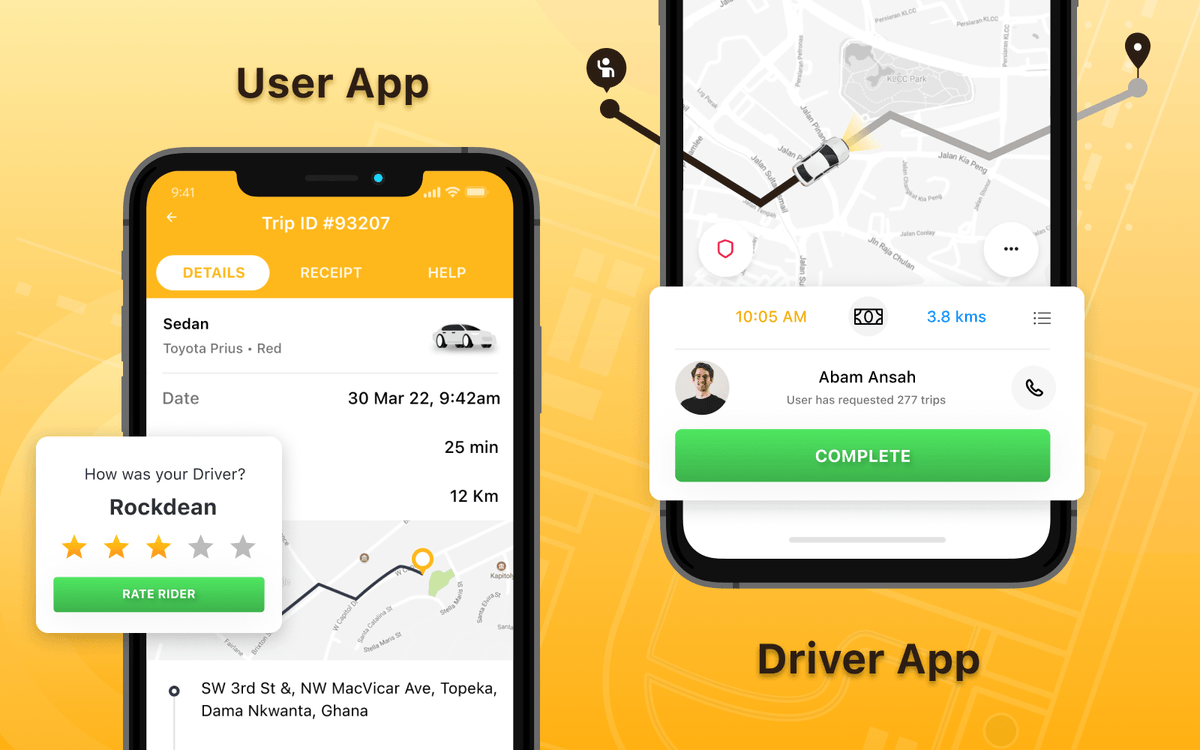The image is a detailed graphic design, likely serving as an advertisement or guide for a mobile application. It prominently features two modern iPhone-like devices, each displaying different screens of the app. The background is a solid golden yellow, providing a vibrant contrast.

**Phone on the Left:**
- The phone has rounded edges and a sleek design.
- At the top of its screen, there is a yellow banner with various buttons labeled 'Details,' 'Receipt,' and 'Help,' along with a heading 'Trip ID 9327.'
- Below, a section displays a trip summary: 'Sedan, Toyota Prius, Red,' followed by the date and time: '30 Mar, 22, 9:42 AM.'
- Further down, it shows travel details: '25 MIN, 12 KM.'
- A highlighted bubble outside the phone provides driver information: 'Rock Dean,' rated '3 stars out of 5 stars,' accompanied by a red 'Driver' button in green.
- At the very bottom of the screen, location details are given: 'SW 3rd Street and NW Viker, Av, Topeka, Dama, NK, Wanta, Ghana.'

**Phone on the Right:**
- This phone is cropped and mainly displays a map with a sedan moving in a zigzag pattern across a monochromatic black, white, and gray backdrop.
- Below the map, another section provides trip details: '10:05 AM,' a dollar symbol indicating cost, and '3.8 KMS.'
- Further information includes the name 'ABAM ANSA' and a profile picture of a man who appears to be of Middle Eastern or Caucasian descent.
- Below the profile picture, it reads 'COMPLETE' within a green button.
- At the bottom of the phone, it reads 'DRIVER APP.'

The overall design is clean and modern, likely aimed at enticing users to engage with the app. The meticulous details and structured information presentation suggest this image is part of a comprehensive guide or advertisement.